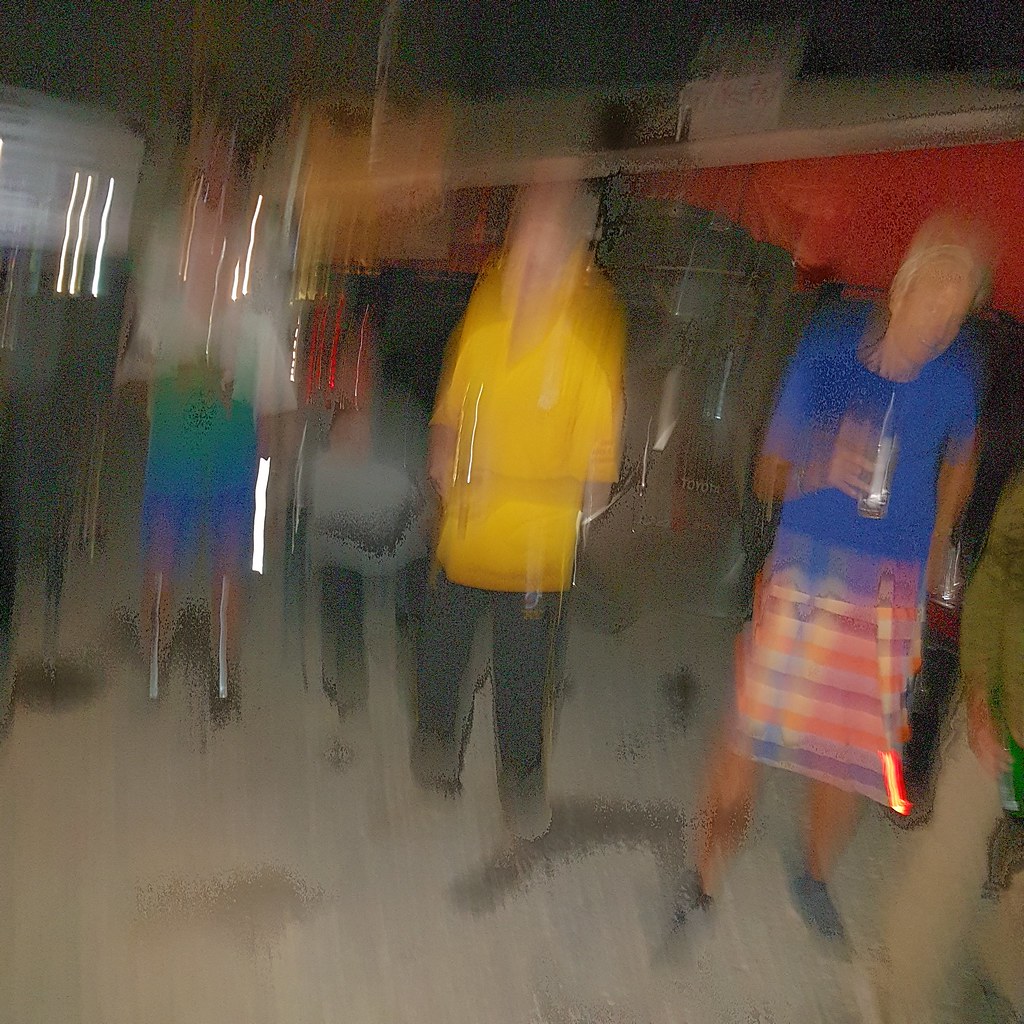This is a very blurry and stretched snapshot taken outside, possibly at a party or a barbecue, featuring a group of people standing in a line on stained concrete, perhaps in a driveway. The background includes what looks like an open garage or a tarp, and possibly a red curtain or banner. Starting from the left, there's a person in blue shorts and a white-to-dark green gradient shirt with an icon on the front, although their face and limbs are not visible due to the blurriness. Next, there is a person sitting or possibly a child in a gray top and black pants, though the stretching makes it hard to discern. In the center, another individual wears a bright yellow short-sleeved shirt with black pants and yellow stripes, appearing to hold something indiscernible. To the right, one person is in a pink, purple, and blue plaid skirt or possibly shorts, paired with a blue shirt, short blonde hair, and seemingly holding a drink. Finally, in the far right corner, an extended arm in a long green shirt is visible. The colors in the photo are distinct, featuring blue, red, yellow, gray, green, white, and brown, contributing to the varied and interesting lighting and shading in the scene.